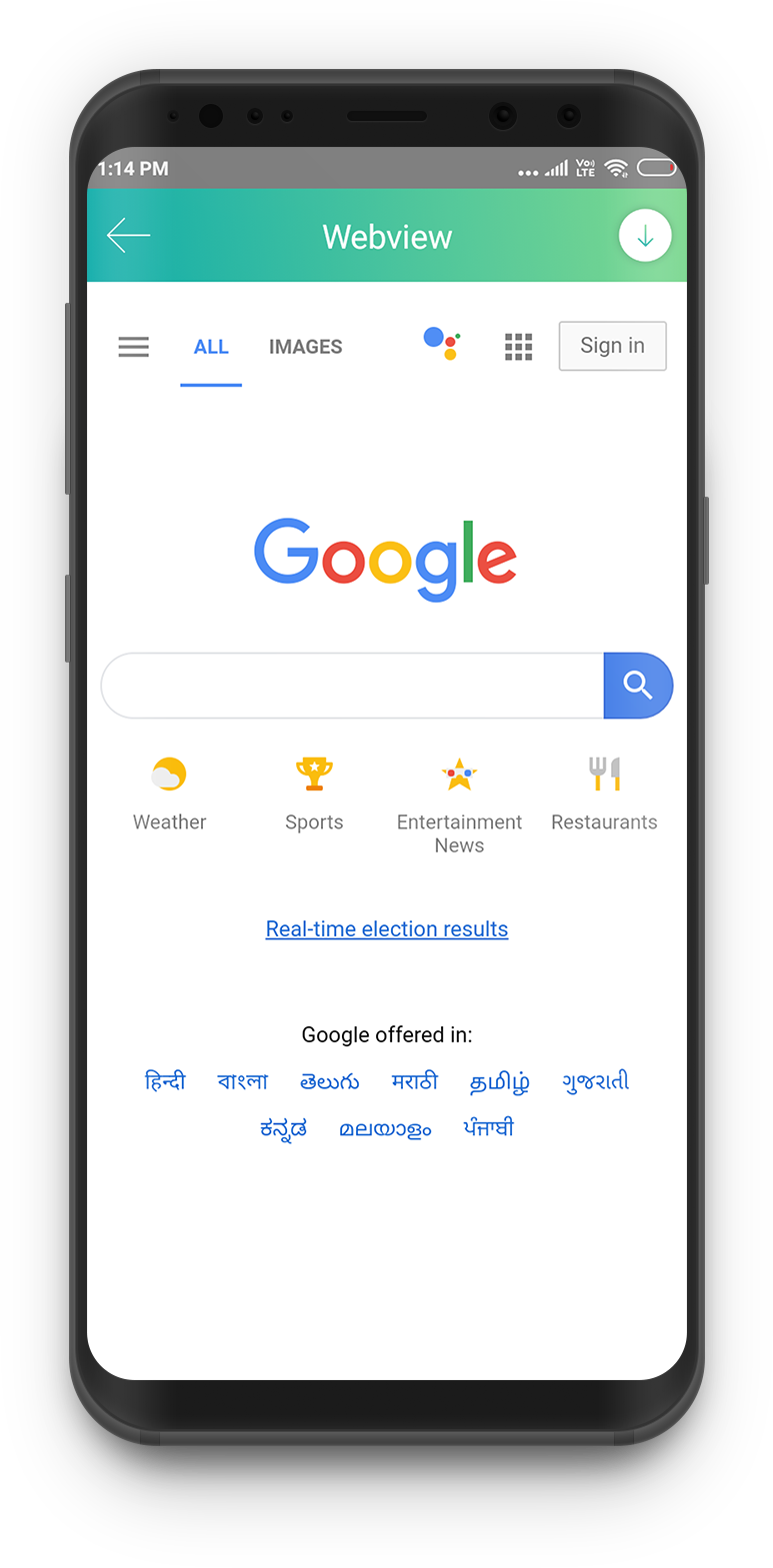The image is a screenshot of a smartphone displaying the Google homepage. At the very top left of the screen, the time reads 1:14 PM. On the top right, icons for data connection, Wi-Fi, and battery status are clearly visible. Centralized at the top, the words "Web View" are displayed. Below this, the navigation options "All" and "Images" appear on the left side, while "Sign In" is placed on the right. Centrally located is the iconic Google logo, vividly colored in blue, red, yellow, and green. Positioned beneath the logo is the search bar. Further down, various category tabs are present, including "Weather," "Sports," "Entertainment," "News," and "Restaurants."